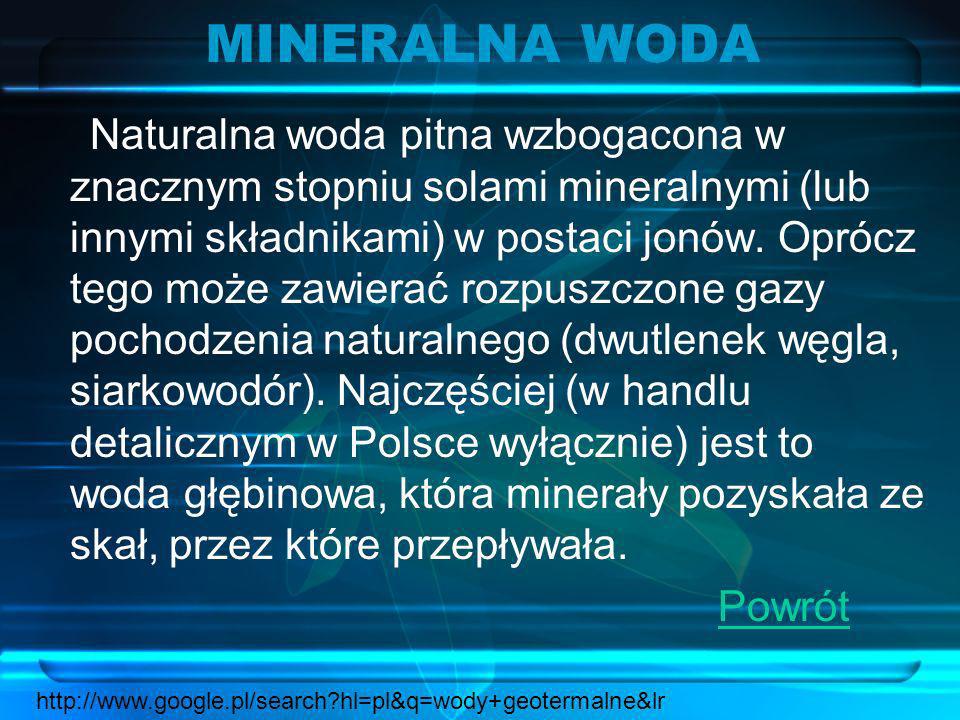The image is a photo of a square screenshot that appears to be a capture of a computer screen with a varying blue background featuring lighter blue swirls and shapes. At the top of the image, in a light blue font against the darker blue background, the title reads "Mineralna Woda" in what seems to be an Eastern European language. Beneath the title is a paragraph of white text written in the same foreign language. In the bottom right corner, the word "Powrot," spelled in green and underlined, signifies something in the same foreign language. Finally, at the very bottom of the image, there is a web address: www.google.pl/search followed by additional letters and numbers.